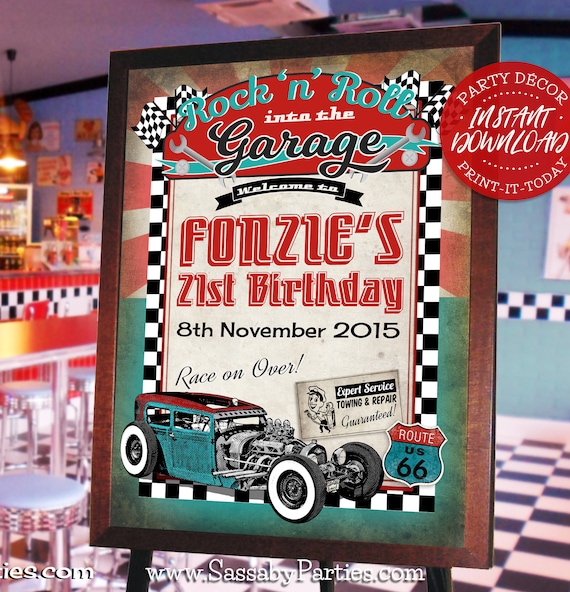This photograph captures a vintage-themed advertisement displayed in a 1950s-style diner. The sign, set in a wooden frame on an easel, reads: "Rock and Roll into the Garage. Welcome to Fonzie's 21st Birthday, 8th November 2015. Race on Over," featuring an illustration of an old-style drag racing car. Additional text includes, "Expert Service, Towing and Repair, Route US-66," and "Party Decor Instant Download Print It Today." The backdrop of the image showcases a classic diner ambiance with a black and white checkered floor, silver bar stools, and a soda fountain. A website, www.sasabeparties.com, is noted at the bottom of the sign, emphasizing customizable party decor downloads available for instant printing.